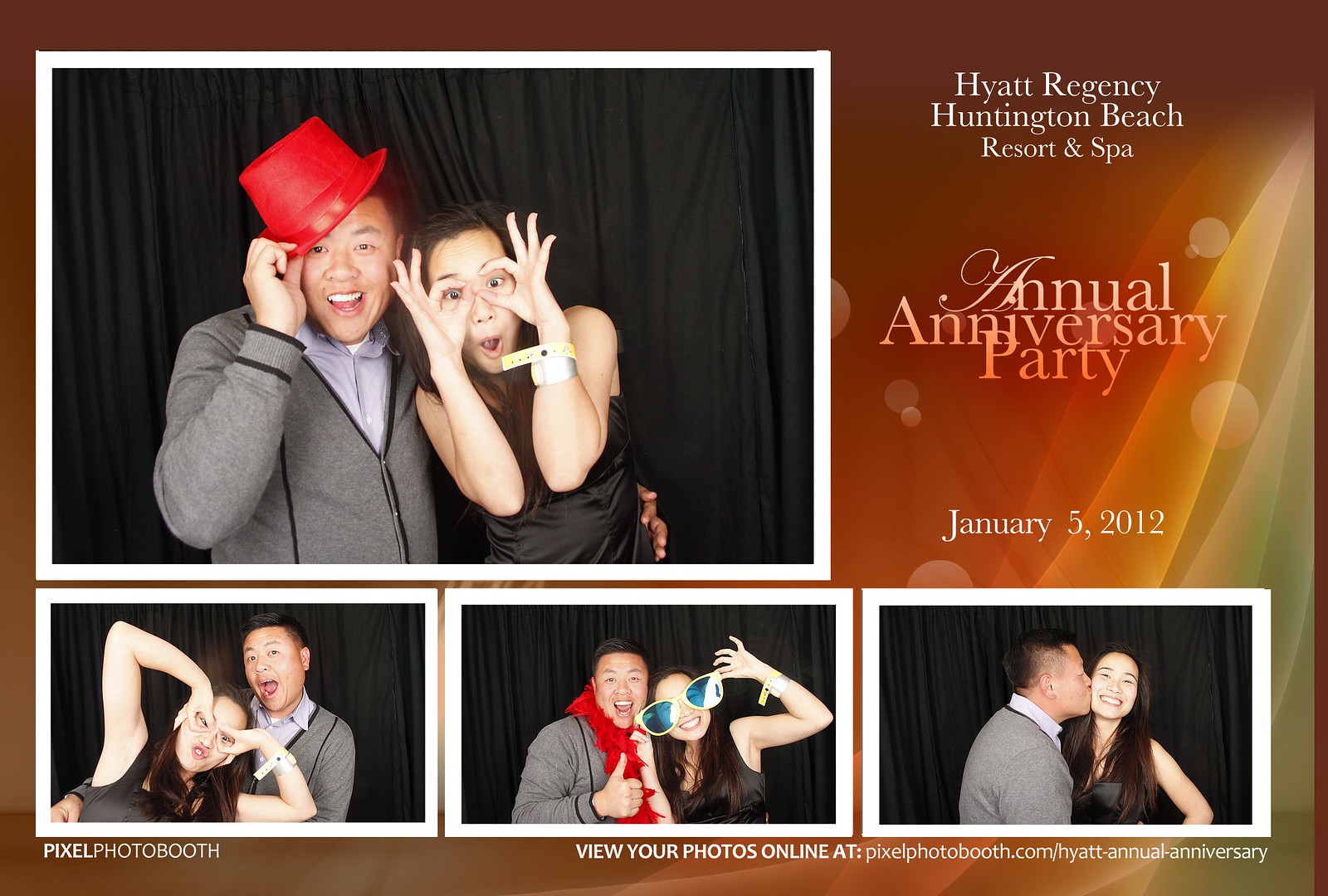### Poster Description: Annual Anniversary Party

**Background:**
The background features a gradient from light brown at the bottom to darker brown at the top, with creamy-colored bubbles scattered throughout. 

**Event Information:**
- **Top Right Corner:**
  - In white print: "Hyatt Regency Huntington Beach Resort and Spa."
  - Below in orange print: "Annual Anniversary Party."
  - Further down in white print: "January 5, 2012."

**Photographs:**
- **Main Photo (Top Left):**
  - A couple is prominently displayed, outlined in white.
  - **Man:** 
    - Wearing a gray long-sleeve shirt with another shirt underneath.
    - Sporting a red top hat, which he's tipping with his right hand.
    - Dark hair, dark eyes, and wide, white-toothed smile.
  - **Woman:** 
    - Long dark hair and dark eyes.
    - Making a 'goggle' gesture with her thumbs and forefingers around her eyes.
    - Wearing a black silk dress and a wristband with a watch.
    - Expression appears surprised.

- **Smaller Photos along the Bottom:**
  1. **Left Photo:**
     - The same man and woman, with the woman repeating the 'goggle' gesture and making a funny face.
     - The man is behind her, laughing, with his mouth open.
  2. **Middle Photo:**
     - The man is now wearing a red fur feather boa, giving a thumbs-up with his mouth open.
     - The woman next to him has put on oversized blue and yellow sunglasses, smiling and holding the side of the glasses.
  3. **Right Photo:**
     - The man is kissing the woman on the cheek.
     - The woman is smiling, showing the right side of her face towards the camera.

**Footer:**
- On the left: "Pixel Photo Booth."
- On the right: "View your photos online at: pixelphotobooth.com/hyattannualanniversary"

This richly detailed caption encapsulates the fun and vibrant spirit of the Hyatt Regency's Annual Anniversary Party, capturing the playful interactions of a couple through a series of whimsical and affectionate poses.